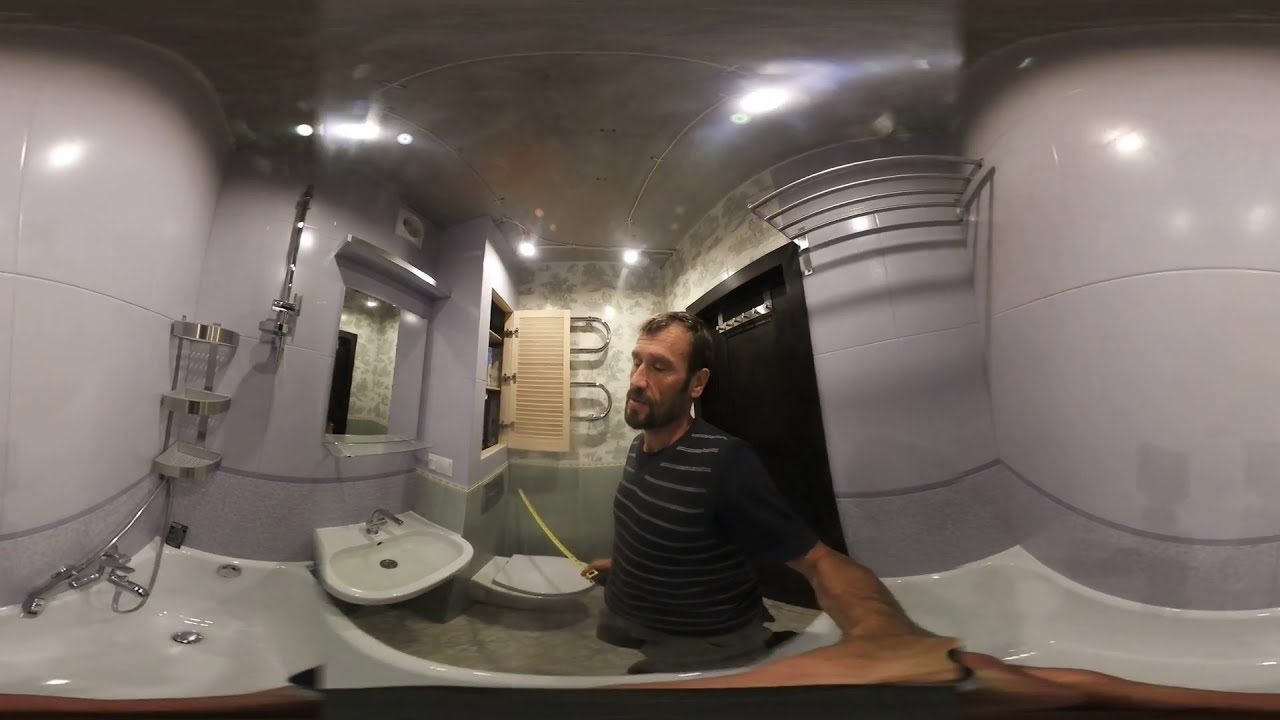The image depicts a man taking a selfie in a bathroom that appears to be undergoing remodeling. He is holding an open tape measure in his hands and is dressed in a black and white horizontally striped shirt with gray shorts. He has a mustache, beard, brown hair with a receding hairline, long ears, and his eyes appear to be partly closed. The bathroom's main colors are grey and white, with the upper walls displaying a grey-lavender hue and white below.

The layout of the bathroom shows a white bathtub with silver railings on the far left and a white sink adjacent to the bathtub. To the right of the sink is the white toilet. Behind the man, there is a black door, and on the right, a wall-mounted silver metal rack likely for towels. In the foreground, the floor is grey and there is a mirror above the sink with three shelves nearby. There is also a cabinet with a shutter door partly open in the middle background. The ceiling is equipped with multiple lights, enhancing the bathroom's modern appearance despite the ongoing construction. The man's relaxed demeanor complements the organized yet unfinished setting.